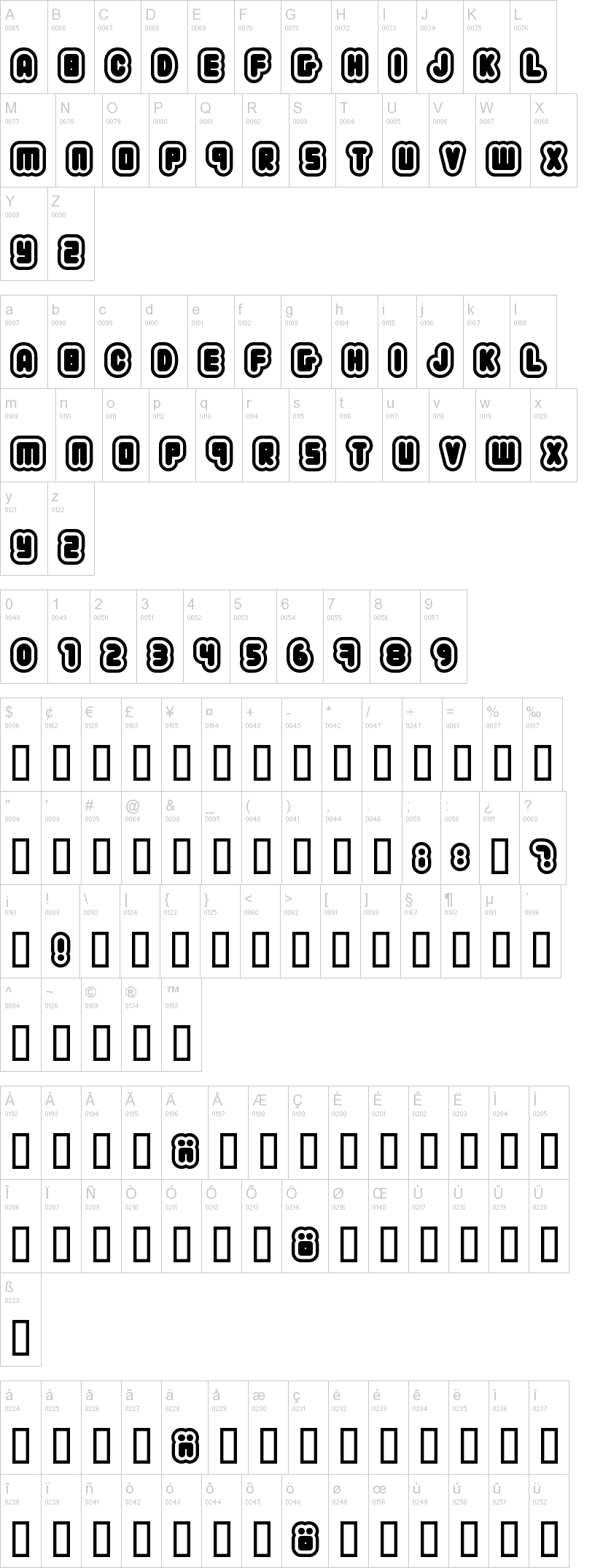The image features a top section displaying letters in bold, shadowed, cartoon-like fonts. The letters are separated into small gray boxes, showing a sequence that reads A, D, C, D, E, F, G, H, I, J, K, L, M, N, N, O, P, Q, R, S, T, U, V, W, X, Y, Z. Each letter is presented in both gray and black-and-white versions.

Below this, a second row showcases the same letters but in a variety of different typefaces. Following the alphabet, there is a series of numbers ranging from 0 to 9. 

Further down, the image presents an assortment of icons reminiscent of those found on cell phones. These include symbols such as bolded eights, a question mark, an exclamation mark, and various camera-like icons. Each symbol is enclosed within a small gray box, separated by gray lines, creating a grid-like structure.

Overall, the image showcases a high-quality design but lacks context, making its purpose somewhat ambiguous.